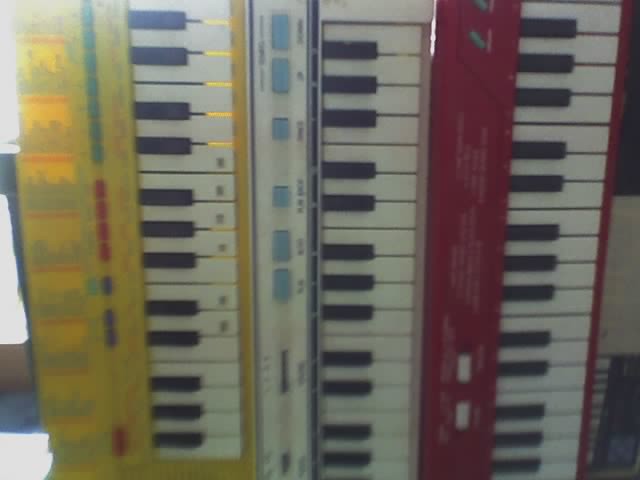The image showcases three vertical electric keyboards positioned side by side against a background with sunlight streaming through a glass door or window, creating a bright, almost washed-out effect. Each keyboard features the customary layout of white and black keys and distinctively colored cases and control buttons. On the far left is a keyboard encased in bright yellow with control buttons in a variety of colors, including purple, red, and turquoise. The middle keyboard has an off-white plastic frame with black and sky blue control buttons. Finally, the keyboard on the far right is housed in a red frame with gray control buttons and notable white text, though it's not legible. The sunlight illuminates the scene from the top left, adding to the vibrant display of colors and textures.